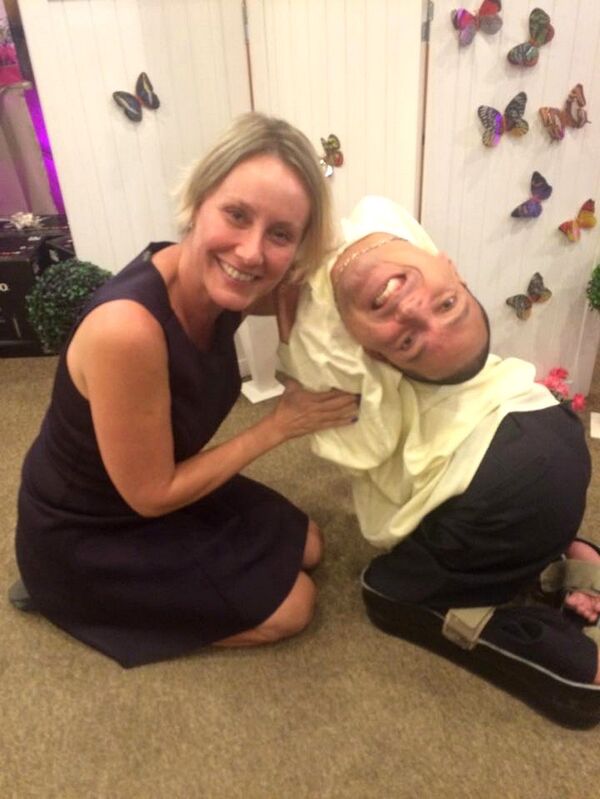In the image, a smiling woman with short blonde hair is seated on a brown carpet, wearing a short sleeveless black dress. She is sitting cross-legged, facing the camera. To her left is a man who appears to have special needs; his head is contorted backwards, giving the appearance of his head being turned in the opposite direction of his body. He is also sitting cross-legged and has no legs, with his limbs positioned on pads on the floor. The man is dressed in black pants and a yellow shirt. The background is a white wood-paneled wall adorned with numerous colorful 3D butterfly decorations. On the left side of the image, a purple light softly illuminates part of the room, enhancing the whimsical atmosphere.